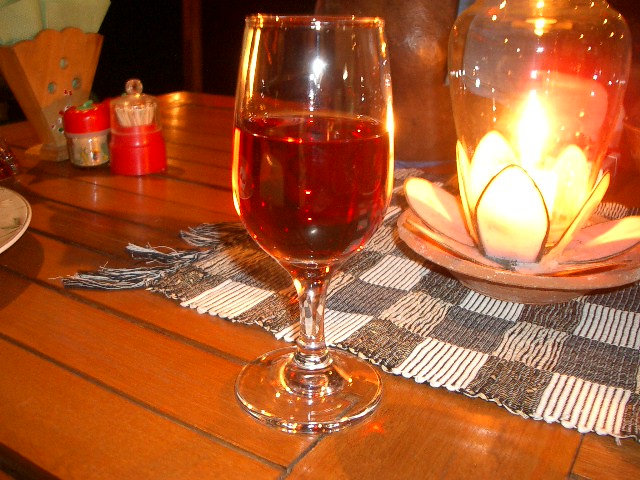The photograph showcases a meticulously arranged dinner setting on a polished wooden tabletop designed to mimic the appearance of planks, with intricate grooves giving it a sophisticated look. Central to the image is a clear wine glass filled with a transparent reddish liquid, gleaming under the light. Adjacent to the glass, a black, gray, and white checkered placemat with frayed edges adds a touch of rustic charm. Resting on the placemat is a brown ceramic dish, beside which sits a vase that doubles as a candle holder; the lit candle inside illuminates the vase, which features a base shaped like a delicate white glass flower. To the left, partially visible are a toothpick holder, napkin holder, and seasoning shaker, contributing to the table's well-set ambiance. The overall scene is a harmonious blend of clear, amber, orange, green, brown, white, black, and gray hues, presenting an inviting and homely dinner table setting.